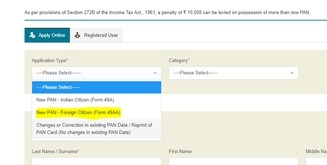The website displayed is challenging to read due to very small text that necessitated zooming in three times, despite the viewer having undergone LASIK surgery indicating the problem is not with their vision. At the top of the website, there's an indiscernible message, followed by a prominent blue line underneath. Directly below the blue line, there are two navigation options: "Apply Online," which is highlighted in blue indicating it is selected, and "Registered User," which is in white and gray. Beneath these options is a drop-down menu that says "Application Type: Please Select," highlighted in blue, though the specific options within the menu are mostly unreadable. Additionally, there is a second highlighted section in yellow, with another unreadable option beneath it. To the right of this section, there is a category option also displaying "Please Select." Below this, an empty white window is present. Under the "Application Type" section, there are fields to enter "Last Name/Surname," "First Name," and "Middle Name," each provided with a white text box for input. All of these elements are set against a beige-colored background, contributing further to the difficulty in readability.